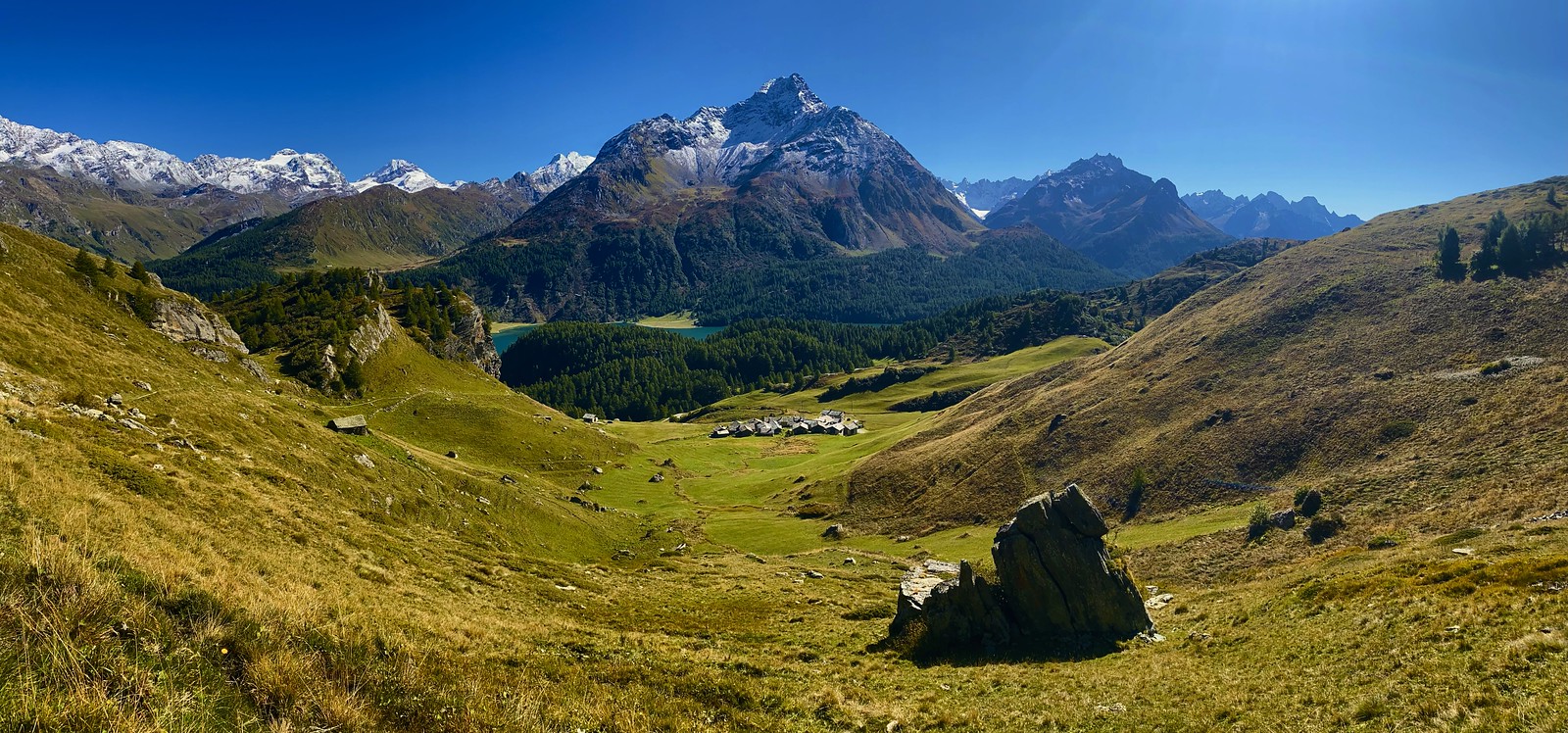The photograph captures a breathtaking valley scene beneath a range of majestic, snow-capped mountains. The foreground features a jagged rock formation surrounded by yellow and light green terrain, with plush green grass and interspersed wild underbrush. The valley curves downwards towards a small, distant village nestled at the base, with tiny houses barely visible. This flat area is flanked by a dense forest of evergreens and pines, giving way to more rocks and patches of greenery. Further down, a serene blue lake lies cradled by the mountains. The valley and hillsides undulate gently, with scattered trees and rock-lined areas adding texture. Above the lush landscape, the towering mountain peaks dominate the scene, their tops blanketed in glistening white snow that may be beginning to melt, signaling spring. The crystal-clear, vivid blue sky stretches above, bathed in radiant sunlight, enhancing the picturesque quality of this serene, sunlit day.